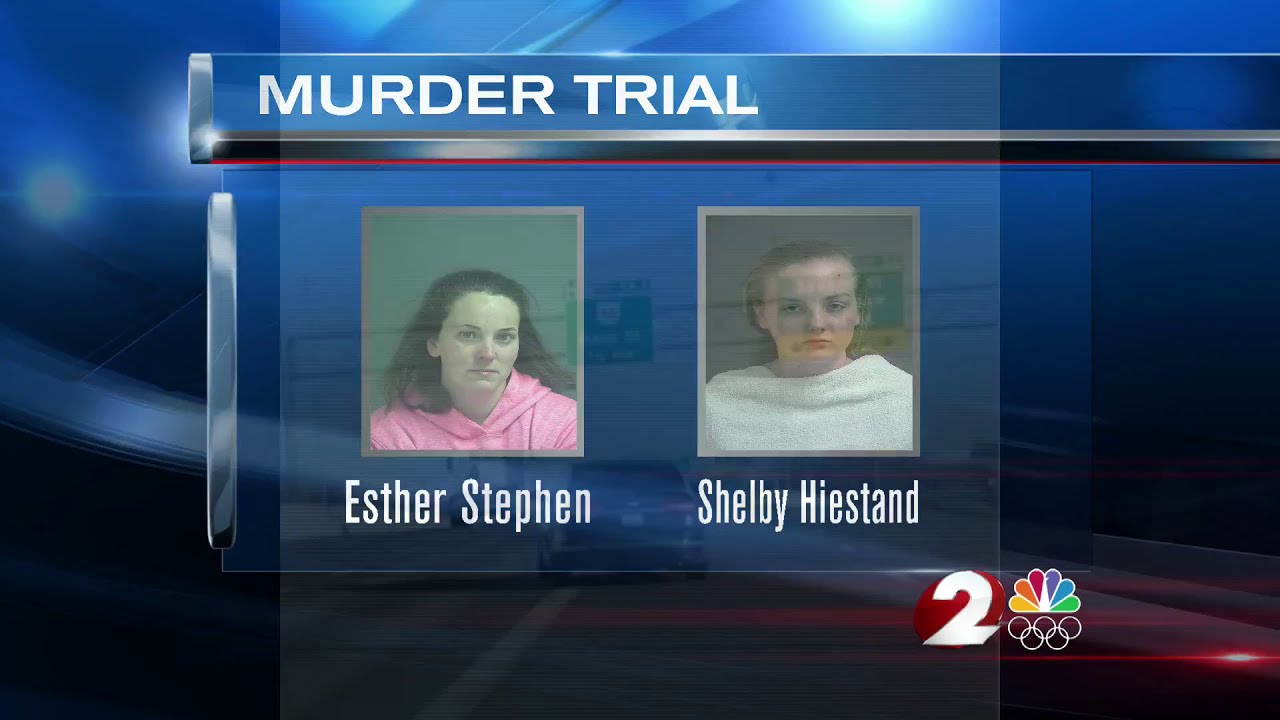The image depicts a still from a local news broadcast about a "MURDER TRIAL," as indicated by the bold white text at the top against a predominantly blue background. Centered below the headline are two photographs placed side by side. The left photograph features Esther Stephen, a white woman possibly in her 30s or 40s, with long dark hair and wearing a pink hooded sweatshirt, her expression serious. The right photograph shows Shelby Heestand, a young blonde woman with shorter hair, donning a white top, also exhibiting a stern expression. Beneath each photo, their respective names are displayed in white text. In the lower right corner of the screen, the NBC Peacock logo with its traditional colors is visible, accompanied by the white Olympic rings and a red circular icon with the number "2" inside, indicating the NBC Channel 2 station logo. The overall background transitions from light to darker shades of blue, adding depth to the graphic.